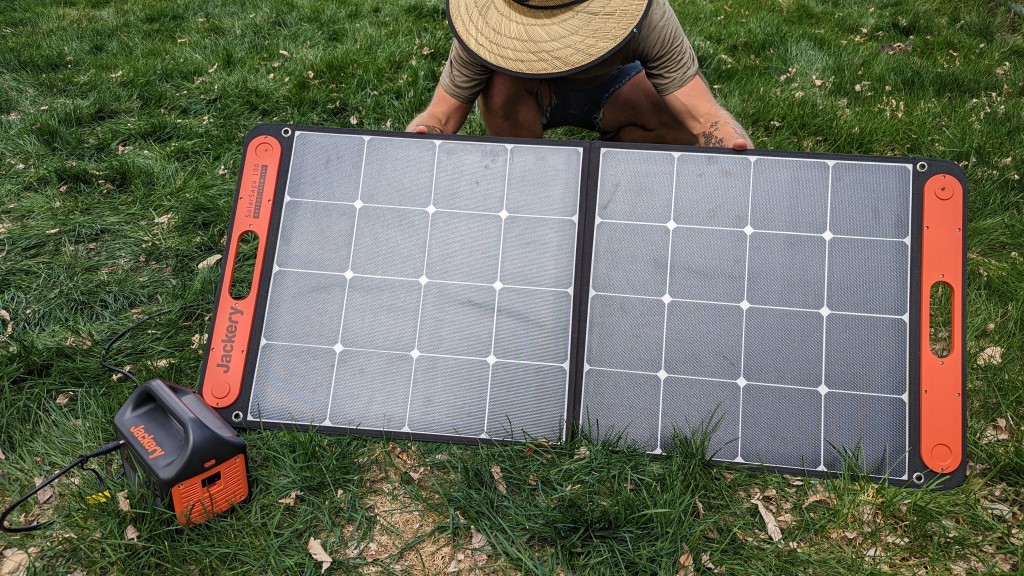The photograph is taken outdoors during the daytime, showing a man wearing a wide-brimmed straw hat and an olive-green t-shirt. He is kneeling on the grass and holding up a large, rectangular object at an angle, suggesting its significant size—approximately five feet long. The object is a solar panel split down the center with a black strip and framed with white lines, creating a grid pattern of light black squares on either side, totaling 16 squares per side. At each end of the panel, there are strips of orangish-red color with oval handholds. The solar panel is labeled "Jackery" and is connected to a small, black portable battery pack that also bears the Jackery name. The setting around the man features green grass dotted with a few brown leaves, indicating a natural, outdoor environment.